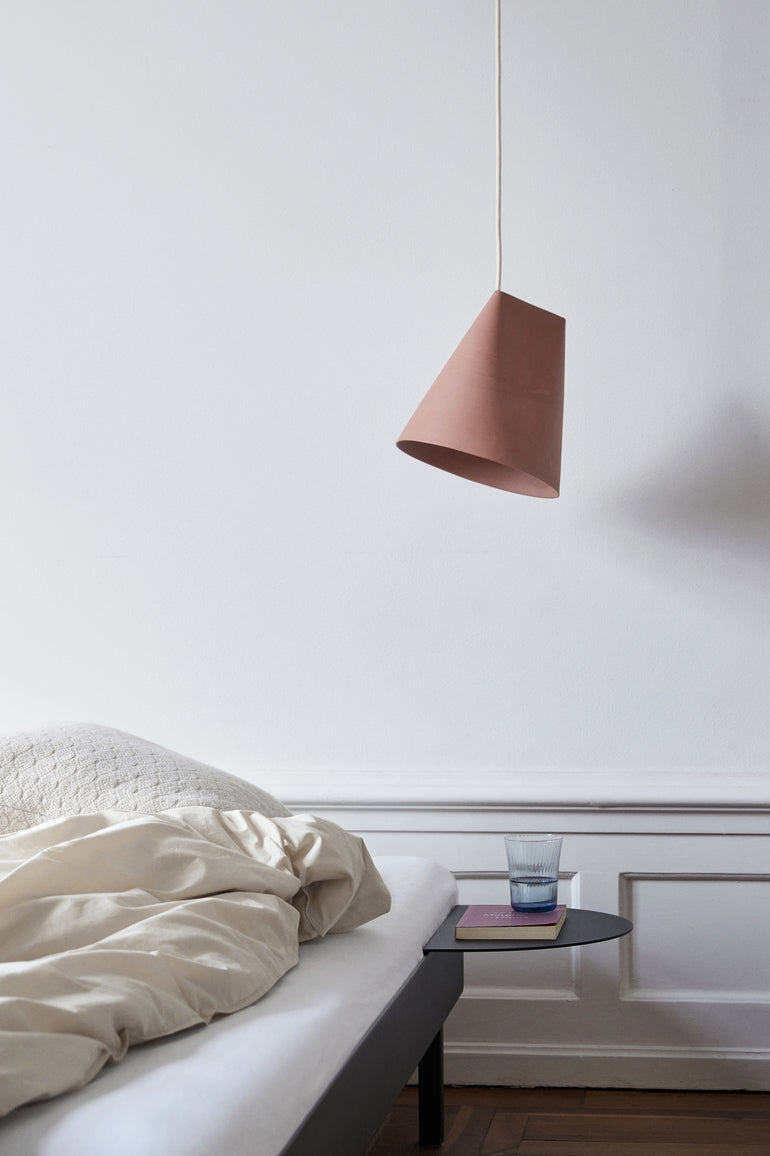This color photograph, captured in portrait orientation, depicts a minimalist bedroom scene characterized by representational realism. The centerpiece of the image is a bed situated in the lower left corner, featuring a thin white mattress adorned with a crumpled beige comforter and a small white pillow. The bed sits on a low black platform with legs, almost flush with the brown wooden floor. Attached to the bed frame is a semicircular shelf serving as a bedside table, on which a blue translucent glass of water and a red-covered book rest. Above this shelf, a distinctive conical purple lamp with a white string hangs from the ceiling, casting light downward and creating a shadow on the right side of the white wall behind the bed. The wall also features white wainscoting at the base. The entire composition emphasizes the central elements: the bed, the glass, the book, and the unique hanging lamp, set against a simple and clean backdrop.